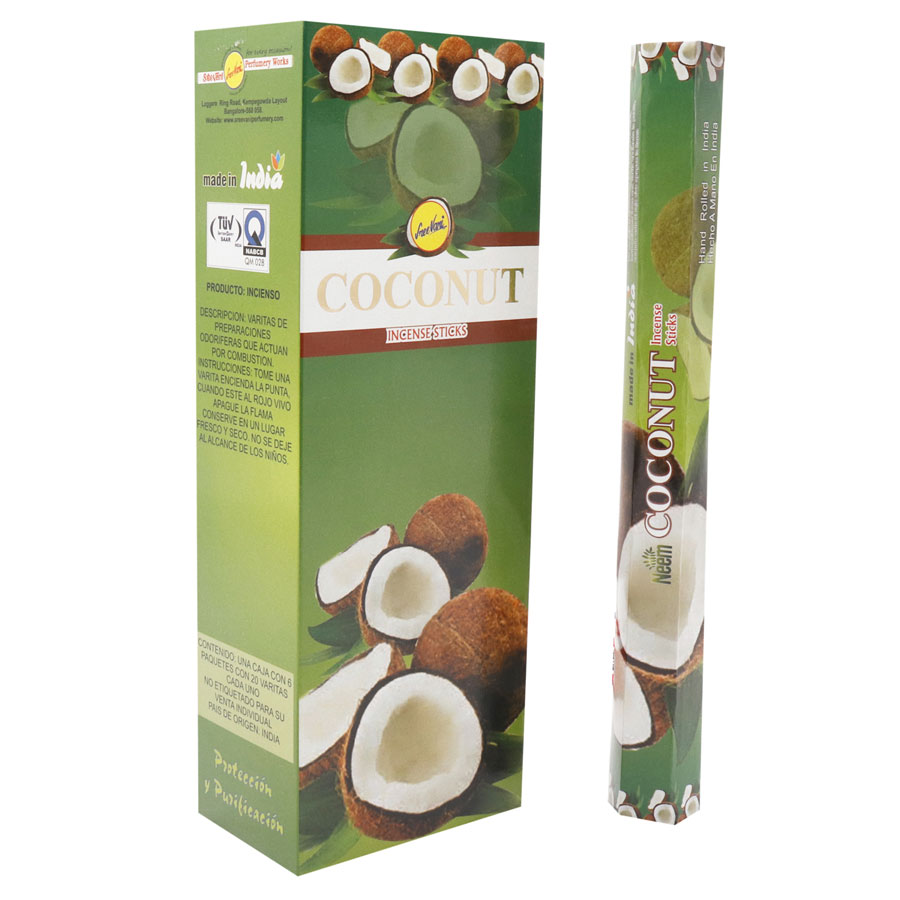This product image showcases a box of coconut incense sticks against a clean, white background. The main focus is on a rectangular, predominantly green box adorned with multiple images of opened and whole coconuts. At the top, the coconut illustrations are repeated four times, with additional, less opaque coconut imagery beneath. The front of the box displays a yellowish logo flanked by green leaves, followed by a series of brown and white lines. The white line bears the word "coconut" in goldish letters, while the bottom brown line reads "incense sticks."

Positioned to the right of the box is one of the coconut incense sticks itself, echoing the same design elements: an image of a broken-open coconut and the words "NEEM Coconut Incense Sticks" written along its side. The box is presented in an isometric view, allowing a glimpse of the side which provides additional product information in a language other than English, including a clear indication that it's "Made in India." This detailed background emphasizes the coconut theme and origins of the product.